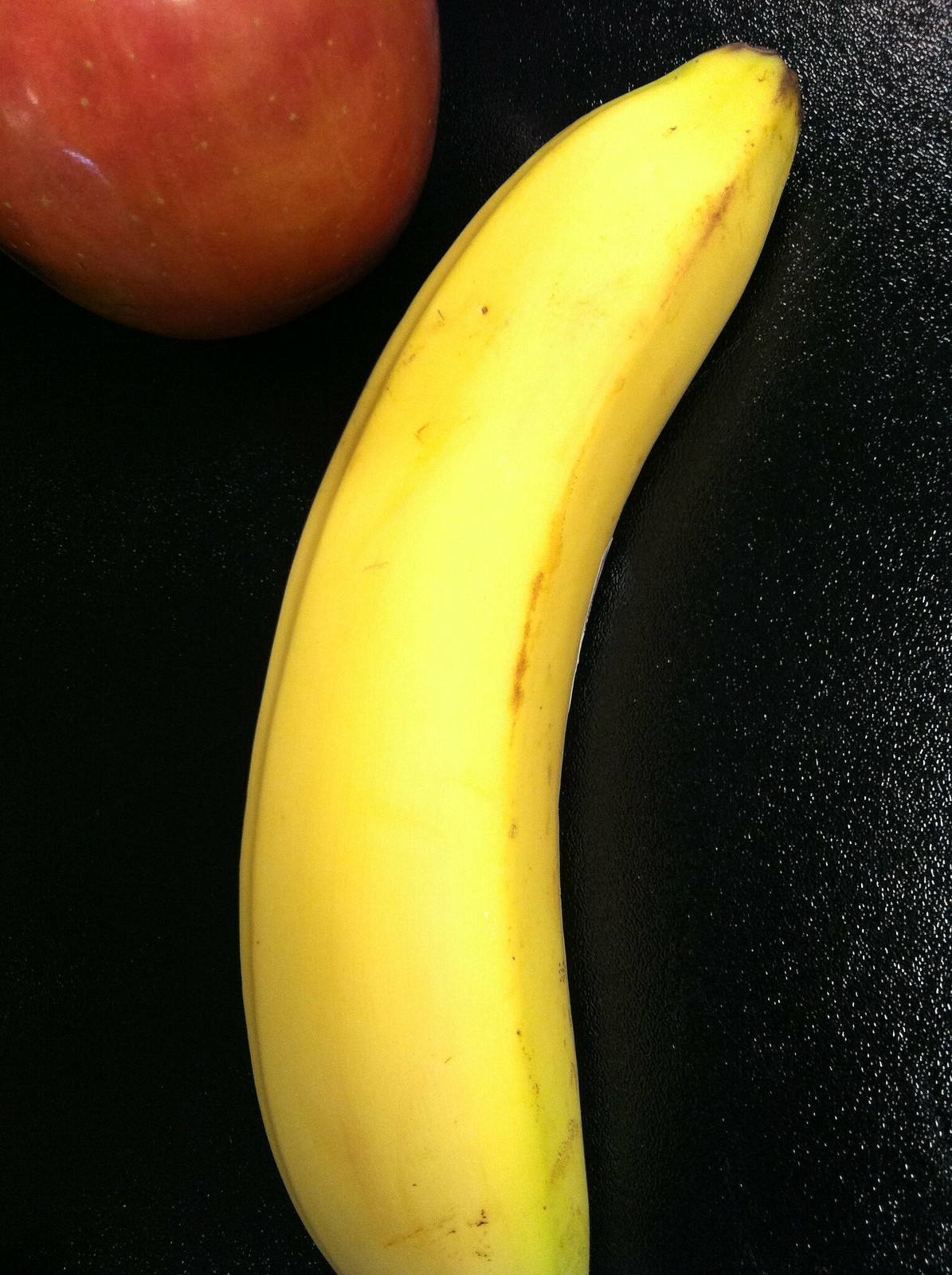Captured in this vibrant photo are two pristine pieces of fruit set against a sleek, black plastic surface that reflects a delicate sheen of light. The first fruit prominently displayed is a banana, still enveloped in its bright yellow peel. Nearly flawless, the peel is smooth with minimal blemishes, featuring just a few tiny brown spots on the curved part of the banana, adding an element of authenticity. The yellow hue is consistent and vivid, with a subtle white reflection indicating the presence of a light source, possibly from the camera flash. Adjacent to the banana is a lustrous apple, its stem hidden from view. The apple's skin is a rich, uninterrupted red, adorned with a sprinkling of natural white specks, enhancing its realistic texture. Together, these two pieces of fruit create a striking contrast against the glossy black background, highlighting their fresh and appealing appearance.